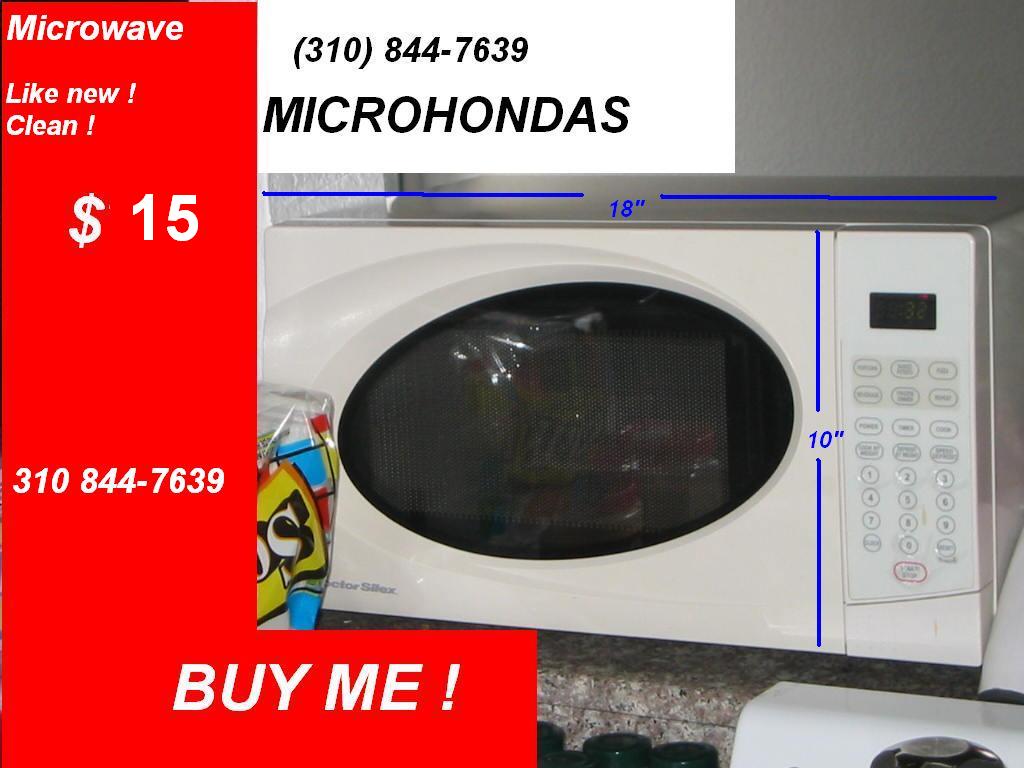The image depicts an advertisement for a used, clean, and like-new white microwave oven for sale at $15. The microwave dimensions are marked with blue lines, indicating it is 10 inches high and 18 inches wide. The appliance features a black oval-shaped window on the door, with standard control buttons to the right. The microwave is placed on a cream and tan tiled countertop, and to the left, there's a red banner resembling a capital "L". The banner displays, in white letters, "Microwave, like new, clean, $15”, followed by the phone number “(310) 844-7639". Below the phone number, it says "Microhondas" in black text. At the bottom of the red section, the words "BUY ME!" are boldly featured in capital letters. Another white rectangle located above the microwave repeats the phone number "(310) 844-7639" along with "Microhondas" below it.